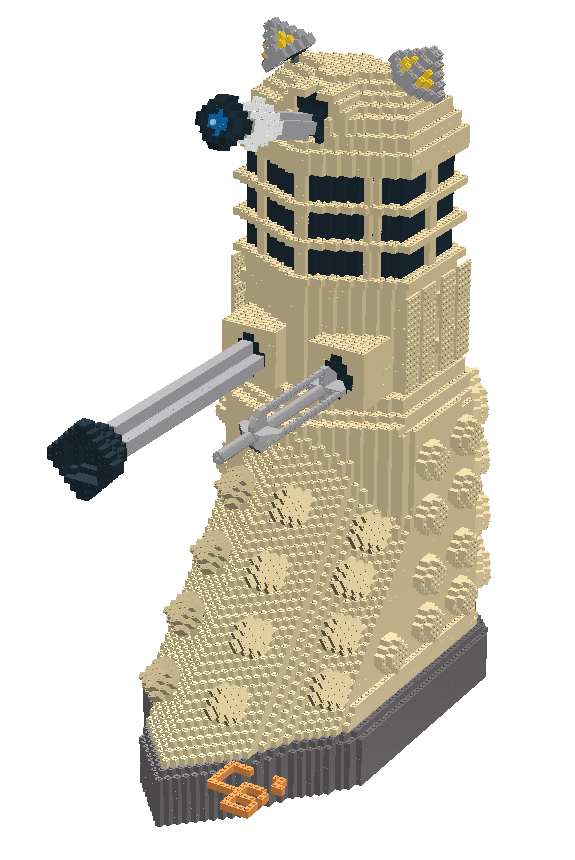The image appears to depict a digitally-rendered, Lego-like structure resembling a tower or fort from a video game, possibly in the style of Minecraft or Sims. The tower is primarily tan-colored with a gray foundation. Near the base, there are prominent bump outs that give the structure a boot-like shape. Just above the gray strip at the bottom, the initials "CB" (or possibly "C8") are prominently displayed in an orange hue. Extending from the front of the tower are two metal prongs, the longer being silver with a black base and the shorter also silver. Higher up, the tower features numerous windows capped by a roof, from which extend two satellite dishes or radar devices that are gray and yellow. There is also a surveillance camera, colored white, black, and blue, emerging from the roof. Additionally, two gun-like turrets, one capped with black, protrude from the middle section of the tower. At the very top, there's another lookout or telescope-like structure. The structure as a whole is intricately detailed, suggesting careful design and construction.